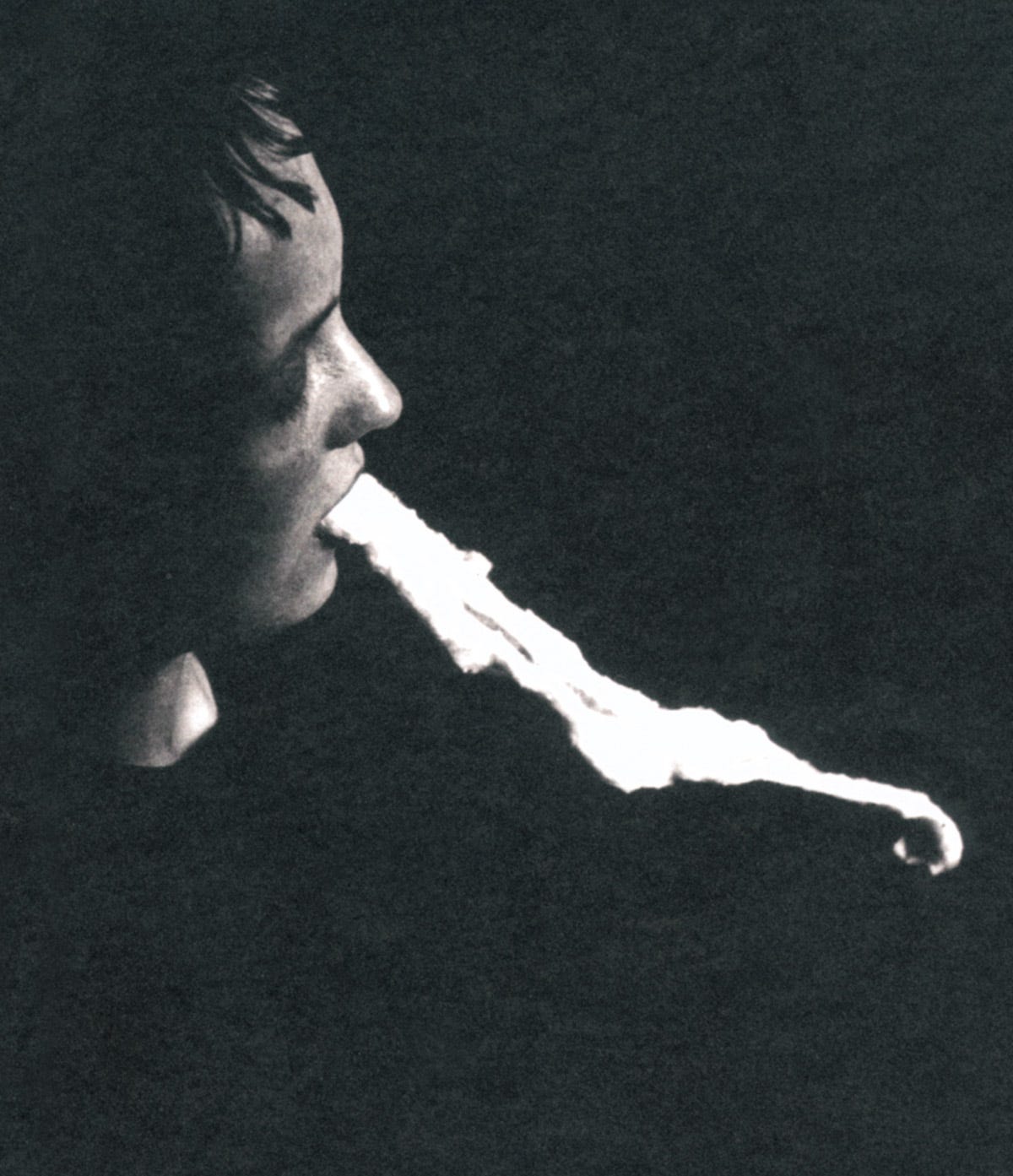The black-and-white photograph, presented in portrait orientation, has a grainy, low-resolution quality that gives it an aged, artistic appearance. The background is completely dark, reminiscent of the graininess one might see when closing their eyes tightly. Occupying the upper left portion of the image is the illuminated profile of a person's face, characterized by dark bangs and black eyebrows, while the right half of their visage and part of their neck emerge from the shadows. The person's mouth is slightly open, from which extends a long, white, tentacle-like object, cutting diagonally across the image and curling towards the bottom. The striking composition, with its surreal and almost ethereal quality, conveys a sense of mysterious motion in the otherwise still and somber scene.